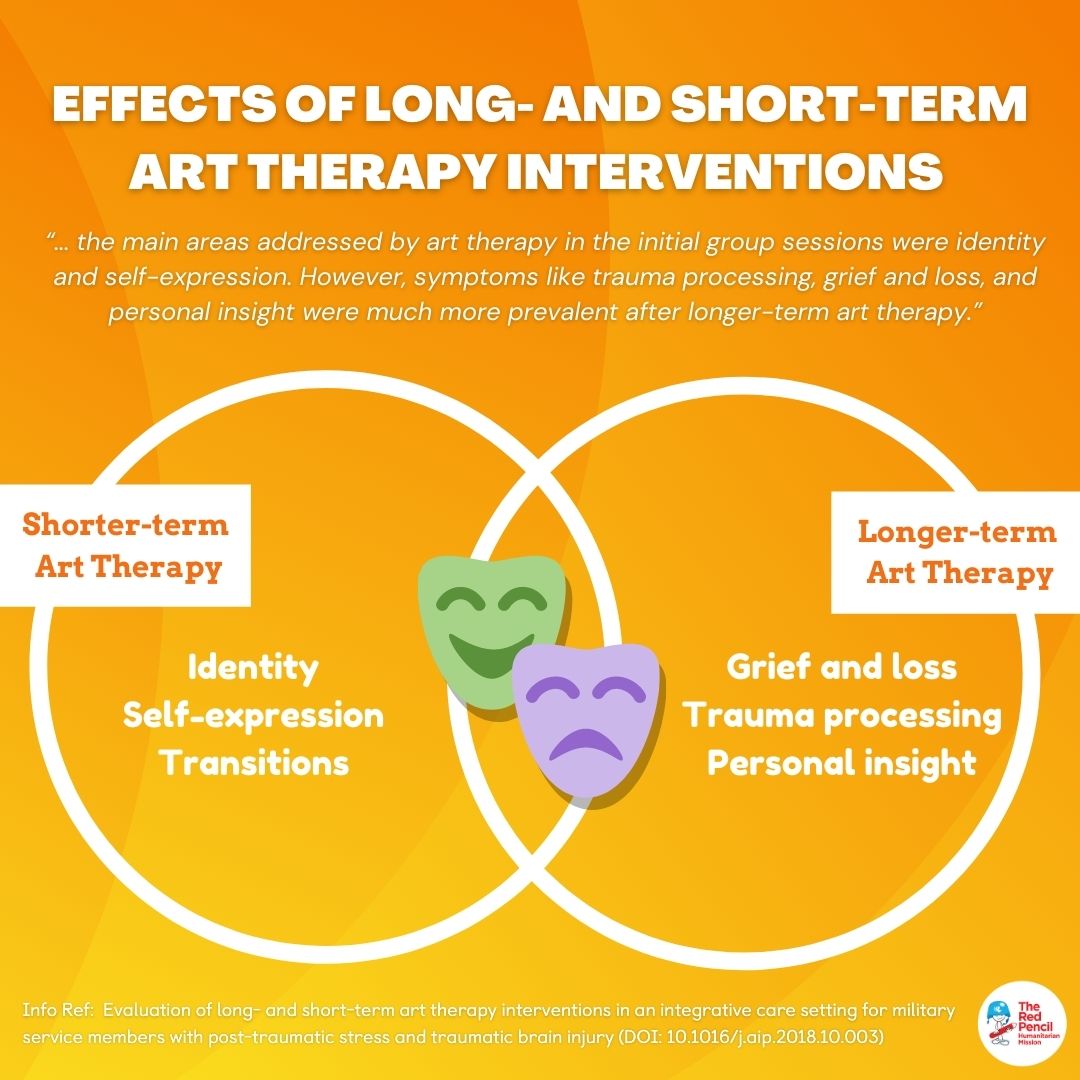This vibrant public service announcement poster uses warm shades of orange and yellow as its backdrop to highlight the transformative effects of art therapy. Across the top, in bold white uppercase letters, it states the "Effects of Long and Short-Term Art Therapy Interventions." Two interlocking white circles sit below, forming a Venn diagram. The left circle, labeled with red text, reads "Shorter-Term Art Therapy" and focuses on identity, self-expression, and transitions. The right circle, labeled in white, reads "Longer-Term Art Therapy" and addresses more complex issues such as grief and loss, trauma processing, and personal insight. In the middle, where the circles intersect, are iconic theatrical masks representing happiness and sadness, color-coded green and purple respectively. This visually engaging poster aims to promote art therapy as a valuable tool for those needing help with self-expression and those dealing with deeper emotional challenges.